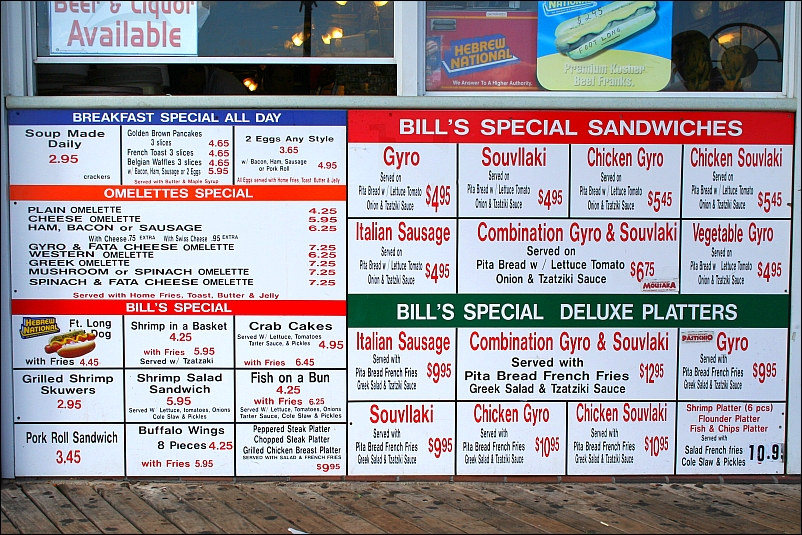A photograph showcases the detailed menu displayed outside of a bustling restaurant, enticing passersby with a wide variety of delicious offerings. The menu highlights an all-day breakfast special, with golden brown pancakes, three slices of French toast, or Belgian waffles, all available with a side of bacon, ham, sausage, or two eggs. For a modest price of $3.65, patrons can enjoy two eggs prepared in any style. The breakfast menu also features an array of omelette specials, including options like plain cheese, ham, bacon, sausage, gyro and feta cheese, western, Greek, mushroom, spinach, and spinach with feta cheese omelettes.

For those seeking hearty options, the menu boasts Bill's Specials, featuring a foot-long hot dog, shrimp in a basket, crab cakes, grilled shrimp skewers, shrimp salad sandwiches, fish on a bun, pork roll sandwiches, buffalo wings (eight pieces), a peppered steak platter, a chopped steak platter, and a grilled chicken breast platter.

Bill's Special Sandwiches section offers enticing choices including gyro, souvlaki, chicken gyro, chicken souvlaki, Italian sausage, combination gyro and souvlaki, and a vegetable gyro. The deluxe platters, listed under Bill's Special Deluxe Platters, consist of Italian sausage, combination gyro and souvlaki, chicken gyro, chicken souvlaki, a six-piece shrimp platter, a flounder platter, and a classic fish and chips platter.

Priding itself on freshly made daily soup for just $2.95, this restaurant clearly caters to a wide range of appetites and preferences, ensuring there is something delectable for every diner who stops by.